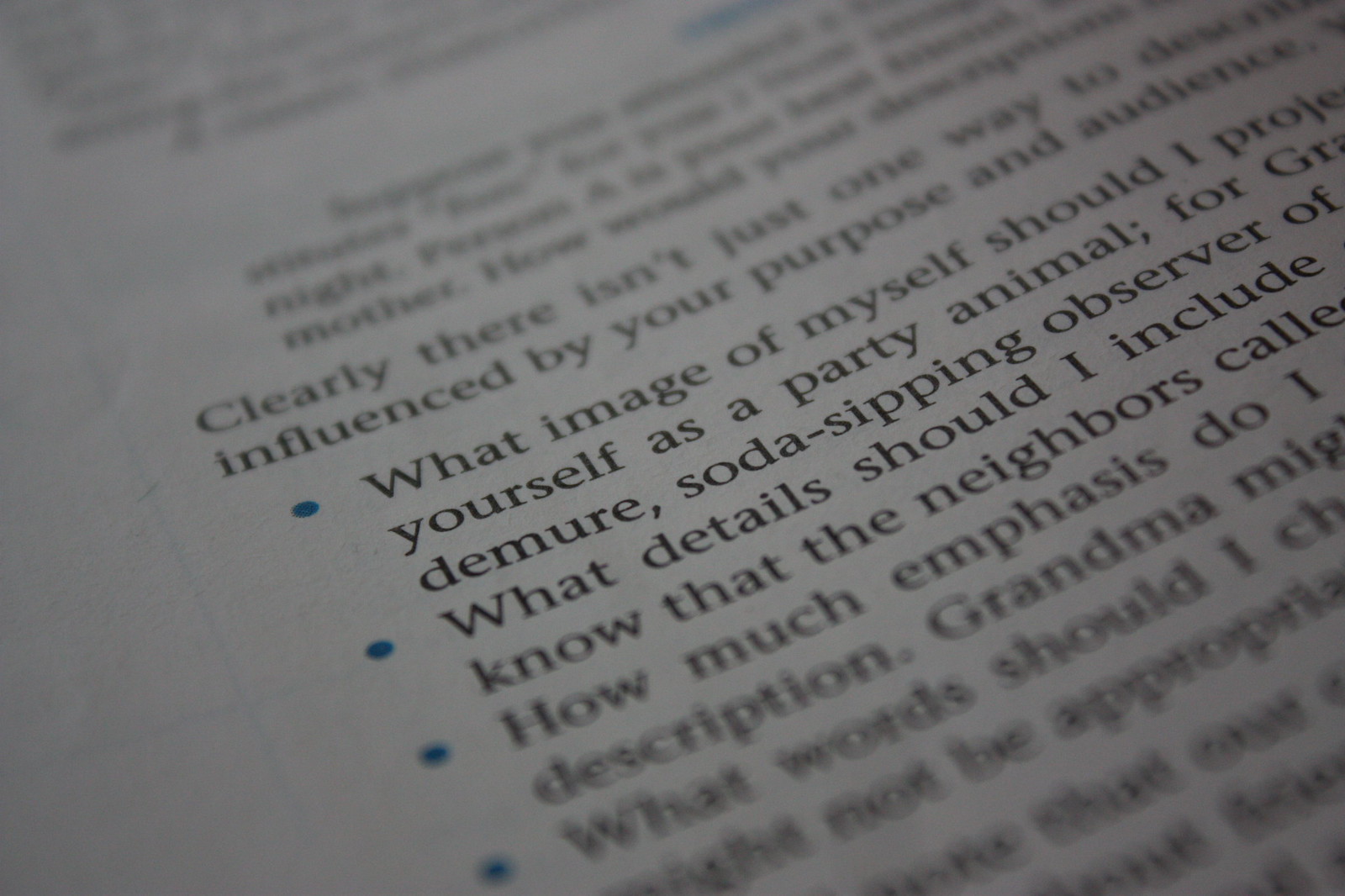The photograph features a close-up of a book page with a distinct white background and black text, accompanied by blue bullet points. The image is tilted approximately 45 degrees counterclockwise, causing the text to appear skewed and partially out of focus, particularly at the top and bottom. Despite this, some text remains legible in the middle portion of the page. The visible content includes: 

- "clearly there isn't just one way to describe,"
- "influenced by your purpose and audience."

Following these lines are several blue bullet points with varying degrees of legibility:

1. "What image of myself should I project?
   - Yourself as a party animal or demure soda-sipping observer of..."
2. "What details should I include?
   - Know that the neighbors called..."
3. "How much emphasis do I..."
   - Description grandma's might..."
4. "What words should I..."

The incomplete sentences and blurred sections indicate that the text continues beyond the visible area, leaving parts of the content cut off and difficult to read.